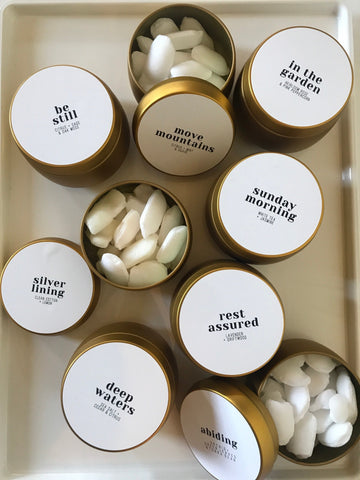An overhead, colored photograph captures the interior of an open box containing an array of small, gold-colored canisters. Each canister is labeled with a white sticker displaying various inspirational phrases in black type. The canisters contain small, white items resembling beans, pills, or possibly bath beads, characterized by their soft, smooth texture with a slightly pointed end, akin to tiny rocks or pieces of chalk. The labeled lids of these canisters read, from top left to bottom right: "Be Still," "Move Mountains," "In the Garden," "Silver Lining," "Sunday Morning," "Deep Waters," "Rest Assured," and "Abiding." Notably, the canisters with the labels "Move Mountains," "Silver Lining," and "Abiding" are open, revealing their contents, while the rest remain sealed, neatly arranged on a white tray beneath them.